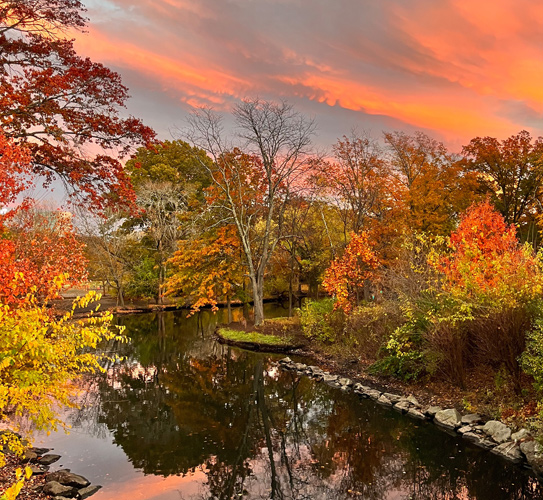The image depicts a serene lakeside or pond scene during autumn, framed by a variety of colorful trees in full fall foliage, including green, red, yellow, and orange hues. Some of the trees already stand bare, creating a picturesque contrast against the vibrancy around them. The calm water, devoid of waves, mirrors the surrounding trees and captures the unique sky above. The sky, with its streaks of bright orange, gray, pink, and hints of purple, suggests the time of either sunrise or sunset. The shoreline is adorned with rocks, and there’s a path visible on the right side, lined with more trees and bushes. The reflections in the clear, clean water enhance the natural beauty of the scene, making it a tranquil and captivating autumn landscape.